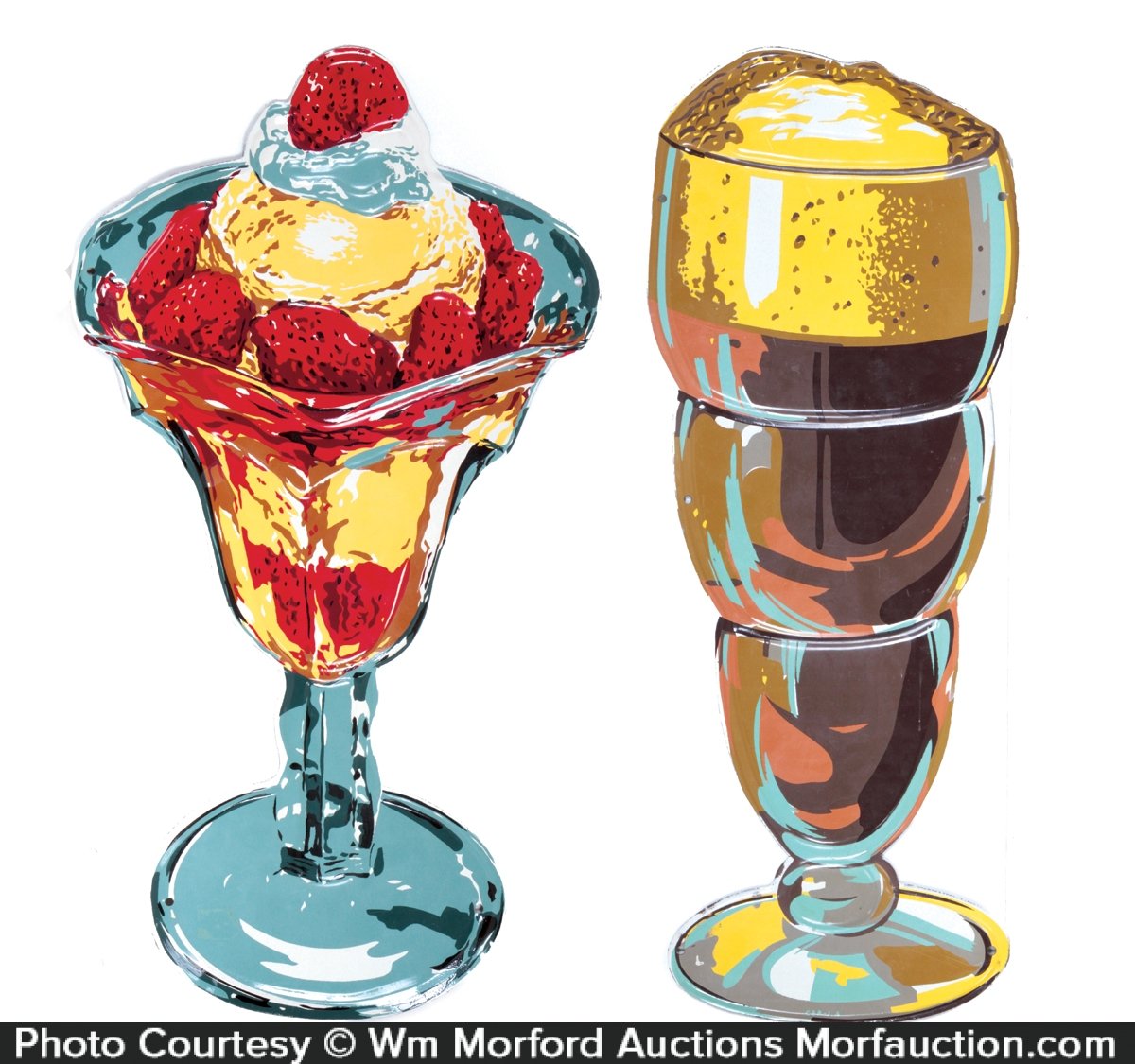The image appears to be an illustration of a dessert menu, set against a white background. On the left side, there is a detailed drawing of a strawberry sundae presented in a clear, blue-tinted glass footed cup. This sundae features a layering of yellow ice cream or custard, topped with a swirl of white whipped cream and adorned with several strawberries, including one placed on the top. To the right, there is another dessert item resembling a root beer float or a chocolate brown soda, characterized by a foamy top and served in a taller, banded glass. Both glasses are illustrated with notable attention to detail, featuring flat bases and progressively widening shapes. At the bottom of the image, a black banner contains the text "Photo Courtesy W.M. Morford Auctions, MorfAuction.com" in white print, despite the image appearing more like a stylized drawing rather than an actual photograph.